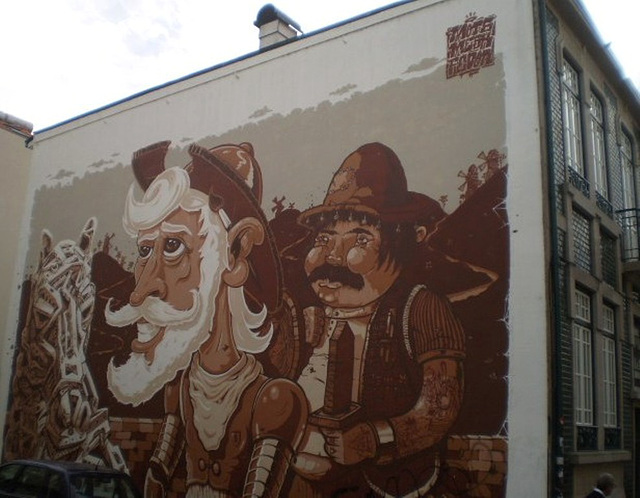This image captures an exterior view of a building framed against an overcast white sky. Most prominently, the photo features an expansive, expertly rendered mural that dominates the side wall of the building. The mural is painted in muted, predominantly brown tones, and portrays two distinct historical figures: 

On the left is an elderly man with dark skin, sporting a white flowing beard and mustache, along with white hair. His head is adorned with a cap that resembles a fireman's hat, which might bear an indistinguishable letter 'R'. His face possesses elongated features with pouches under his softly expressive green eyes, a distinguished white handlebar mustache, a big white crescent-moon-shaped chin, and a nose that is slightly elongated. He’s wearing what appears to be knight's armor paired with a white scarf, possibly symbolizing Don Quixote with a calm, introspective demeanor.

To his immediate right stands a robust middle-aged man also of a darker skin tone, featuring short black hair and a pronounced black mustache. He is dressed in a brown hat, short-sleeved brown shirt, and brown vest with hints of white. He holds a wooden sword in his left hand, with a lively jasper-like expression and generously round features, portraying a jovial attitude somewhat reminiscent of a sidekick or follower. His facial details include tiny eyes, a slight pouting lip, and a rounded jawline.

Further to the right of the mural, one can see what appears to be a horse adorned in white armor, decorated with intricate zig-zag patterns, enhancing the historical and adventurous theme of the mural.

In the background of the depiction, a winding path can be seen curving into a distant mountain range. Adjacent to the mural, partially visible is the connected front of the building, characterized by traditional architecture with dark green facade, flat roof, and rows of multi-pane windows across two levels. 

The mural is rich in detail and artistic skill, melding humor with historical reference, suggesting a narrative that uniquely combines elements of Western and historical themes, possibly hinting at a modern retelling of Don Quixote's adventures.